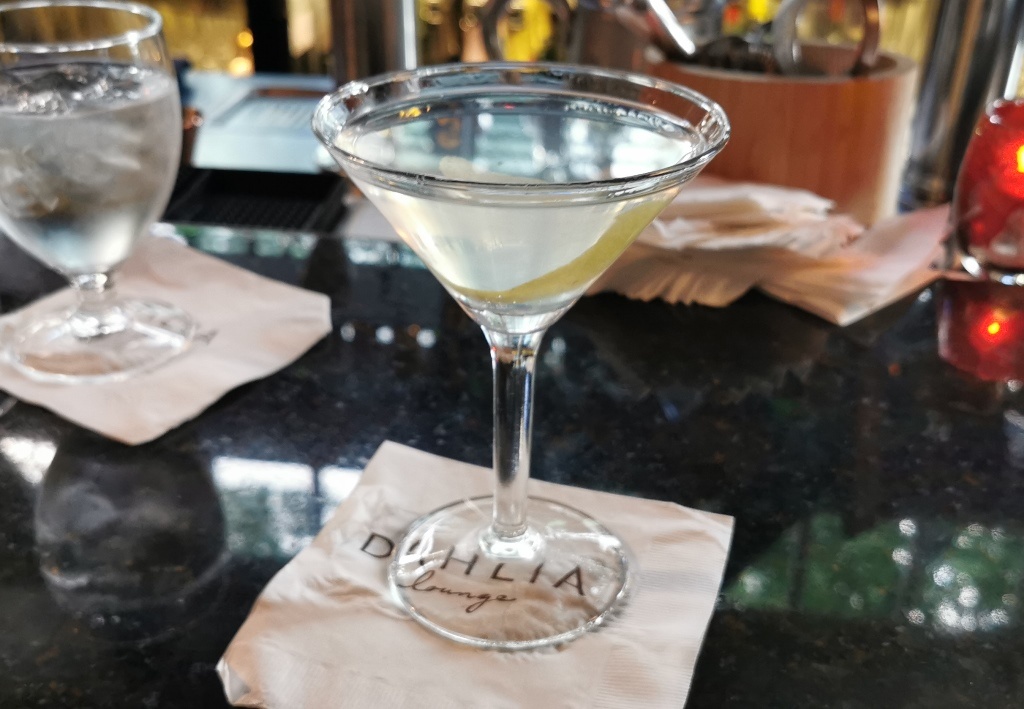In this detailed digital photograph, we see a close-up of a sophisticated bar counter with a reflective, marbly texture. Dominating the center of the image is a brown paper napkin with the words "DAHLIA LOUNGE" printed on it in black text, the latter portion in cursive. On this napkin, a clear wine glass filled with a yellow, apple cider-colored liquid takes center stage, indicative of some type of alcoholic beverage, potentially a margarita. To its left, there's a normal water glass also positioned on a Dahlia Lounge napkin. The right side of the image features what appears to be a candle, contributing to the intimate ambiance. Behind the wine glass, additional napkins are visible along with a beige, cylindrical wooden container that could be a knife rack. The overall scene is set against a backdrop of blurred elements, suggesting additional bar equipment and glasses, adding to the luxurious and inviting atmosphere of the Dahlia Lounge.